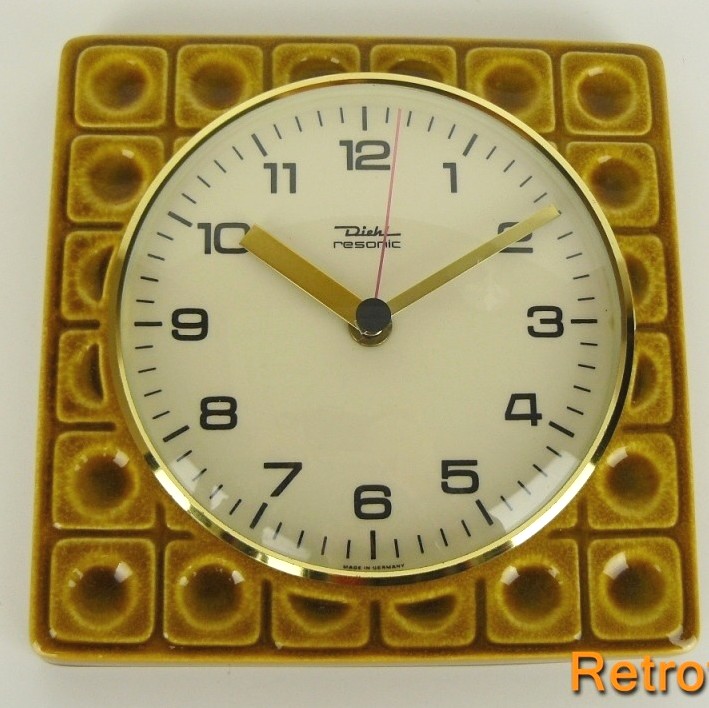This photograph captures a retro-style clock mounted on a wall, blending vintage charm with intricate design details. Positioned prominently in the image, the clock features a striking white face with clear black numerals, accented by precise black markers for accurate time-telling. The hour and minute hands are crafted from a gold or brass-colored metal, adding a touch of elegance, while the vibrant red second hand creates a bold contrast as it rests between the two and three-second marks, indicating 10 minutes past 10.

Surrounding the clock face, a circular metallic ring with a golden or bronze finish enhances the timeless appeal of the piece. This central element is encased in a unique square frame, which appears to be made from high-fired porcelain or clay. This frame is decorated with a grid of smaller squares, each featuring a central round circle, adding texture and depth to the overall design.

In the lower right corner of the photograph, the word "retro" is prominently displayed in orange letters, reinforcing the nostalgic aesthetic. The meticulous combination of materials and design elements makes this retro clock a captivating focal point against the wall.